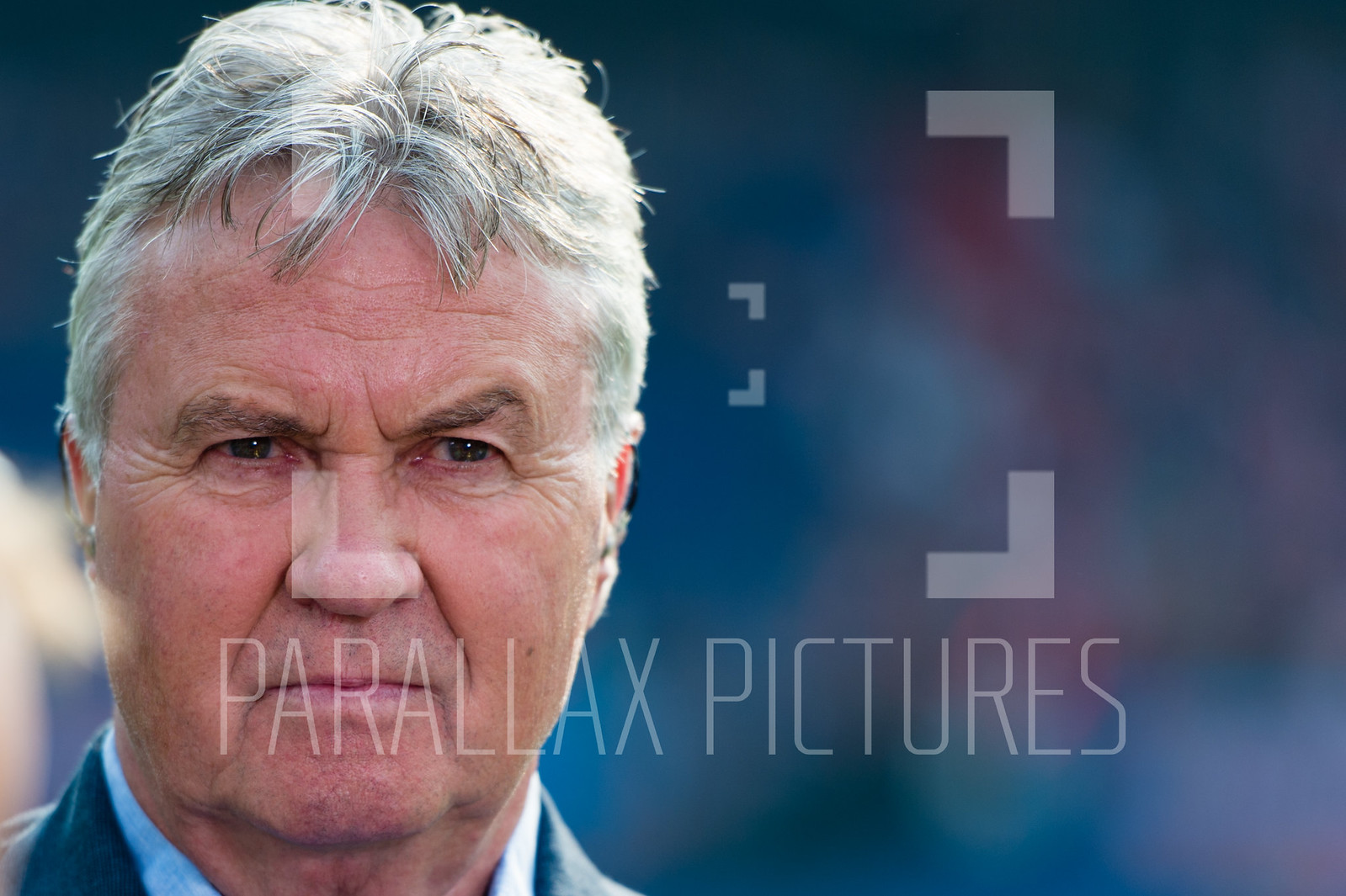This close-up image features an older white man with predominantly grey, slightly messy hair with hints of black. He has a tan-pinkish complexion and deep laughter lines around his nose. His eyebrows are black and scrunched, contributing to a pronounced frown, and his lips are set in a tight line. His forehead and the area between his eyes are wrinkled, and he has crow's feet at the corners of his eyes, giving him a stern, possibly judgemental expression. He appears to be wearing a navy suit jacket over a white collared shirt, though only his neck and a bit of his collar are visible. The image background is an indistinct blur of blues and reds with hints of purple and yellow, likely from a glare. Overlaid on the photo, slightly below the center, is a clear grey watermark that reads "Parallax Pictures" with a square icon above the text. The man appears unimpressed, adding a layer of intensity to the portrait.